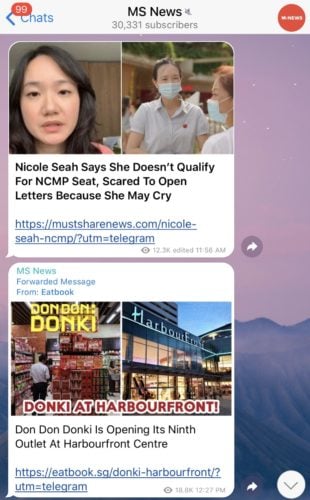The image in question is a vertically oriented rectangular graphic positioned at the top center of a white horizontal background. At the top of this vertical image, the text "MS News" is prominently displayed in black font, with "M" and "S" capitalized. Directly below this heading, in light gray font, it states "30,331 subscribers."

On the upper left corner of the white background, the word "chats" appears in blue font, accompanied by a left-pointing arrow. A small red oval with the number "99" in white font overlaps this section. To the right, there is a red circle with indiscernible content inside.

Moving leftwards, the graphic does not extend to the edge, and houses a vertical rectangular area featuring two stacked images. The top image displays an Asian woman, while the image beneath shows two women wearing face masks. Below these images, black text reads: "Nicole Sia says she doesn't qualify for NCMPC, scared to open letters because she may cry." A blue hyperlink is situated directly underneath this text.

In a second rectangular section further down, on the upper left corner it reads: "MS News forwarded message from Eatbook" with "MS News" in green font and the rest of the text in blue. This section contains two side-by-side images. The left image appears to be set in a grocery store with yellow signage that reads "Don Don: Donki." The right image depicts an area resembling a store, with "HarbourFront" written on it. Overlaying both images, in bold red font on a white background, is the caption: "DON DON DONKI AT HARBOURFRONT!" The accompanying text below announces: "Don Don Donki is opening its ninth outlet at HarbourFront Centre," followed by a web address.

Surrounding these vertical rectangular posts on the right side, the background features a gradient transitioning from a lighter purple at the top to a darker purple at the bottom.